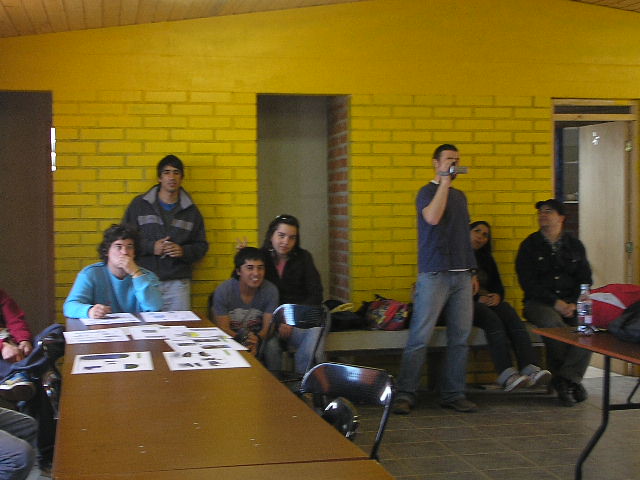The photograph captures a lively scene of young adults congregated in a room with a distinctive yellow-painted brick wall, revealing glimpses of its original red brick around a doorway. The setting includes a variety of seating and tables, creating a dynamic environment.

Toward the right, an open wooden door with a light brown frame adds to the room's character. In the foreground on the left, two long folding tables with wooden tops and black legs are arranged together, displaying multiple white pieces of paper with pictures. Surrounding these tables are black folding chairs, two of which are occupied by partially visible individuals seated at the far left edge of the photo.

The center of attention is a group of young adults who seem captivated by an off-screen event. Leaning against the yellow wall is a gentleman in a gray windbreaker. In front of him, a boy in a blue sweatshirt sits at the table, adjacent to another boy in a gray sweatshirt. Next to him, a girl with sunglasses perched on her head, dressed in a black jacket, playfully gives bunny ears to the boy in the gray sweatshirt as she looks directly at the camera. Close by, another young man in a gray shirt and blue jeans holds up a camcorder, documenting the scene, drawing the curious gazes of two more people to his left. 

On the table in front of this group, various items including a red backpack, a brown backpack, and a bottle of water are scattered. The intriguing composition and the array of candid poses highlight the engaging moment shared among these young adults in this detailed and colorful setting.